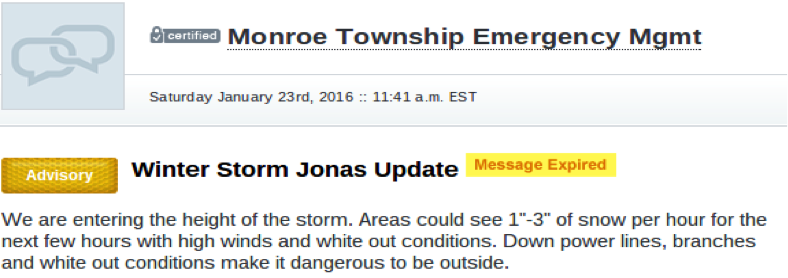The webpage shown is the official site of the Monroe Township Emergency Management Department. At the top, a prominent headline reads "Monroe Township Emergency Management." Adjacent to this headline on the left-hand side, there's a labeled box that says "Certified," signaling the authenticity and official status of the page.

The webpage also displays the exact date and time: "Saturday, January 23, 2016 at 11:41 a.m. Eastern Standard Time." Immediately below, under a distinct "Advisory" headline encased in a yellow box, the alert "Winter Storm Jonas Update" is announced. Accompanying this, another yellow box with orange lettering indicates that the message has expired. The advisory message details, "We are entering the height of the storm. Areas could see 1 to 3 inches of snow per hour for the next few hours with high winds and whiteout conditions. Downed power lines, branches, and whiteout conditions make it dangerous to be outside."

Overall, the webpage is designed to convey urgent and critical information regarding the severe weather conditions posed by Winter Storm Jonas, emphasizing the significant hazards and advising caution.